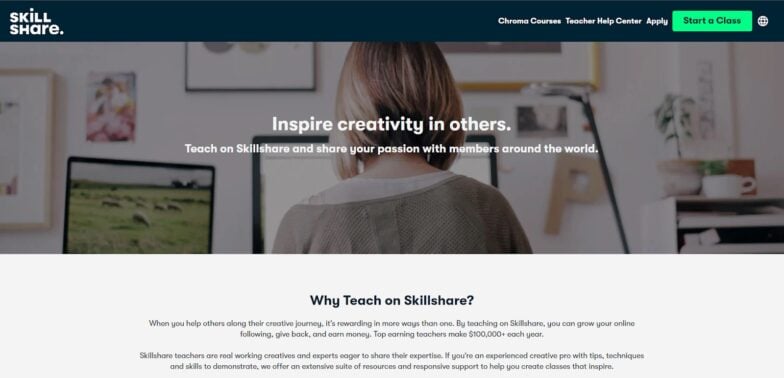The image showcases a woman with the text emphasizing the benefits of teaching on Skillshare, an online learning community. The prominent features include calls to inspire creativity in others, teach on Skillshare, and share your passion with a global audience. Key elements displayed are the Skillshare logo, a green rectangle with the phrase "Start a Class," and a globe icon, symbolizing the worldwide reach of the platform.

The text encourages users to join Skillshare as a teacher, highlighting the motivational phrase "Why Teach on Skillshare?" in blue. It further elaborates on the rewarding aspects of helping others on their creative journeys. By teaching on Skillshare, individuals can grow their online following, contribute to the community, and earn money, with top teachers making over $100,000 annually. The image also underscores that Skillshare teachers are real, working creatives and experts passionate about sharing their knowledge.